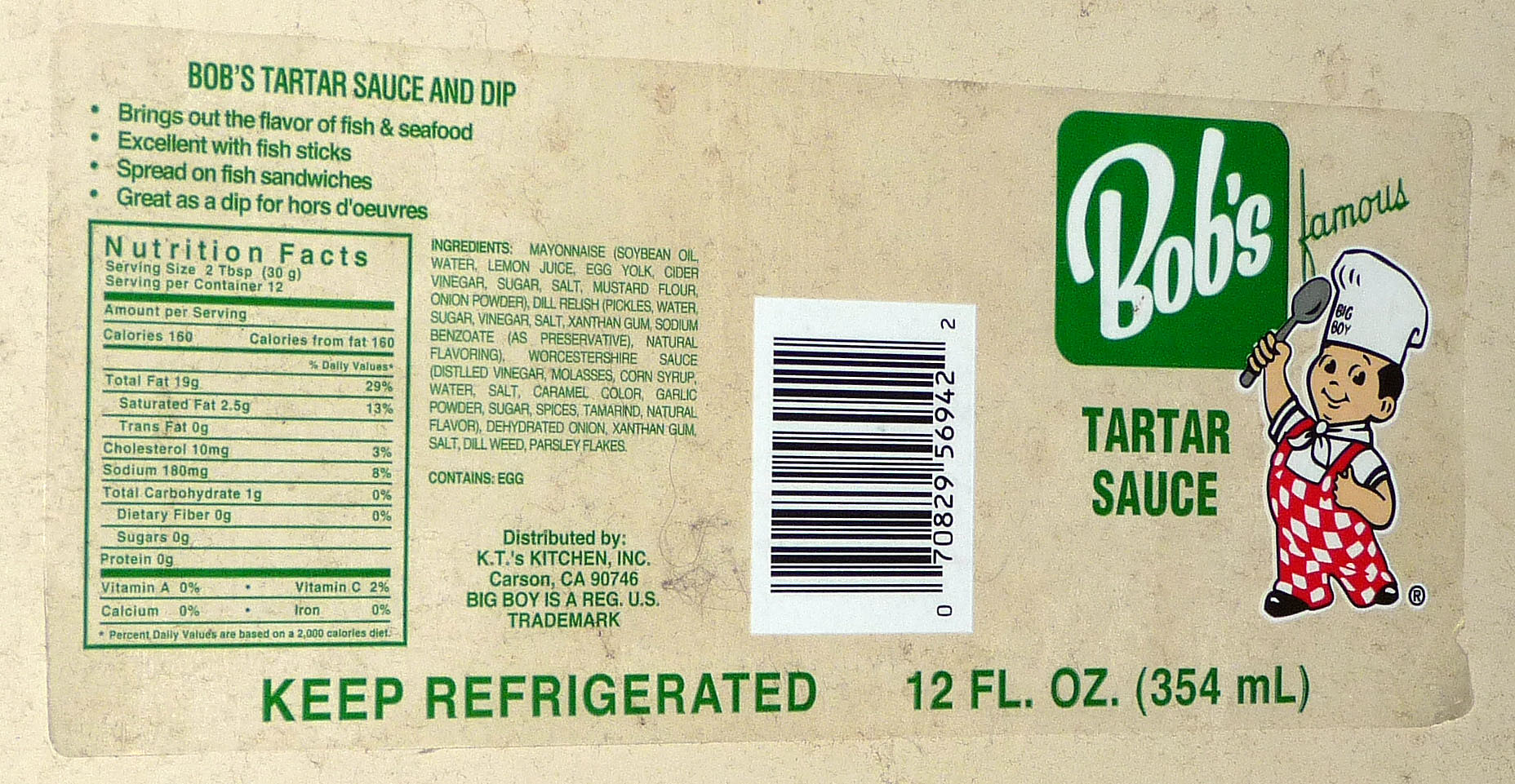The label for Bob's Famous Tartar Sauce features a nostalgic cartoon of the Bob's big boy mascot, characterized by his black hair, white skin, and outfit consisting of red and white checkered overalls, a chef's hat emblazoned with "big boy", and black shoes. The brand name, "Bob's Famous Tartar Sauce," is prominently displayed on a green sign with white lettering. The label includes key product details: 12 fluid ounces (354 milliliters) and a directive to "keep refrigerated" at the bottom. In the center, a barcode is present. To the left, a description reads, "Bob's Tartar Sauce and Dip brings out the flavor of fish and seafood. Excellent with fish sticks, spread on fish sandwiches, great as a dip for hors d'oeuvres." The right side of the label hosts a comprehensive nutrition facts panel and an ingredients list. The product is distributed by KT's Kitchen Inc., Carson, California, 90746, and mentions that "big boy" is a regulated US trademark. The background of the label has a sandy tan color, enhancing the vintage feel of the design.